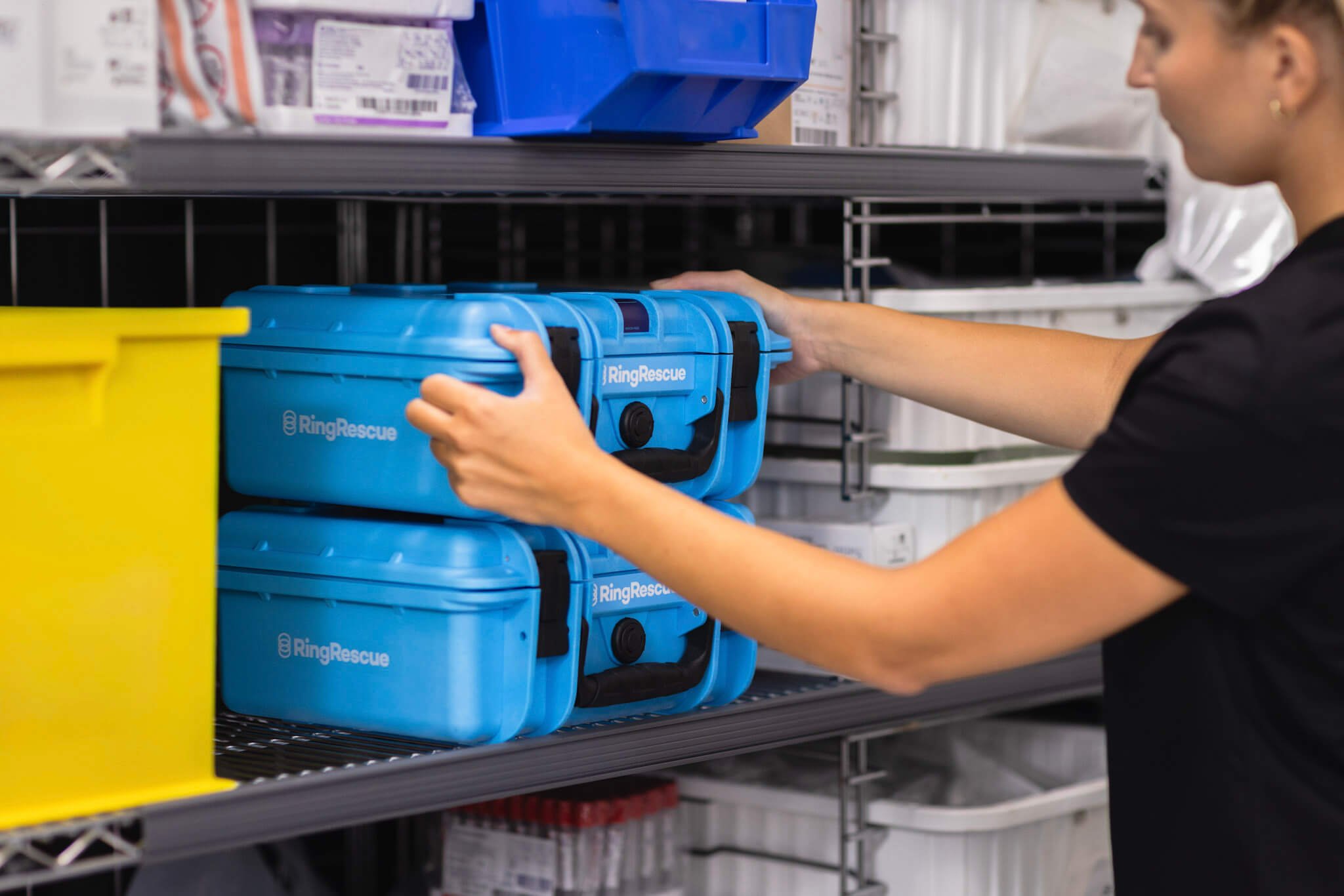A photograph captures a woman with short brown hair wearing a black short-sleeve shirt and earrings, positioned on the right side of the image. She is facing left, with her hands extended toward a blue container labeled "Ring Rescue" in white fondant, which she is either picking up or placing on a metal shelf. The photo is taken indoors, revealing multiple rows of metal shelves laden with numerous white bins, a couple of blue bins, and a yellow bin. The shelf immediately beneath the ones she's handling holds a collection of syringes. The woman appears to be engaged in an activity related to the "Ring Rescue" product, possibly promoting its use. The top half of her body and head are partially cropped out of the frame, drawing attention to her interaction with the blue case, which has a dark handle and is situated on the center left of the image.